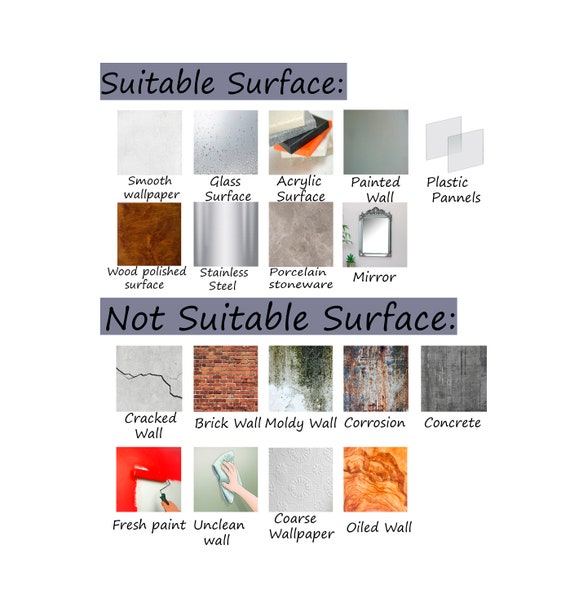This detailed guide provides a comprehensive overview of suitable and unsuitable surfaces for a specific application, likely related to printing or adhesion. At the top, a prominent header labeled "Suitable Surfaces" introduces a series of visuals, each depicting a different type of surface. These visually represented surfaces are meticulously labeled as follows: smooth wallpaper, glass surface, acrylic surface, painted wall, plastic panels, wood polish surface, stainless steel, porcelain, stoneware, and mirror. 

Each image under the "Suitable Surfaces" section is accompanied by a clear indication that these surfaces are appropriate for printing, likely highlighted by the word "print" at the bottom of each picture.

Beneath this, another section titled "Not Suitable Surfaces" provides a contrasting list of surfaces that are inappropriate for the same application. This section, equally detailed, includes individual images of each surface, labeled as cracked wall, brick wall, moldy wall, corrosion, concrete, fresh paint, uncleaned wall, cork wallpaper, and a boiled wall. 

The guide effectively uses a combination of visual aids and text to convey which surfaces are appropriate and inappropriate for specific tasks, ensuring clarity and ease of understanding for the viewer.